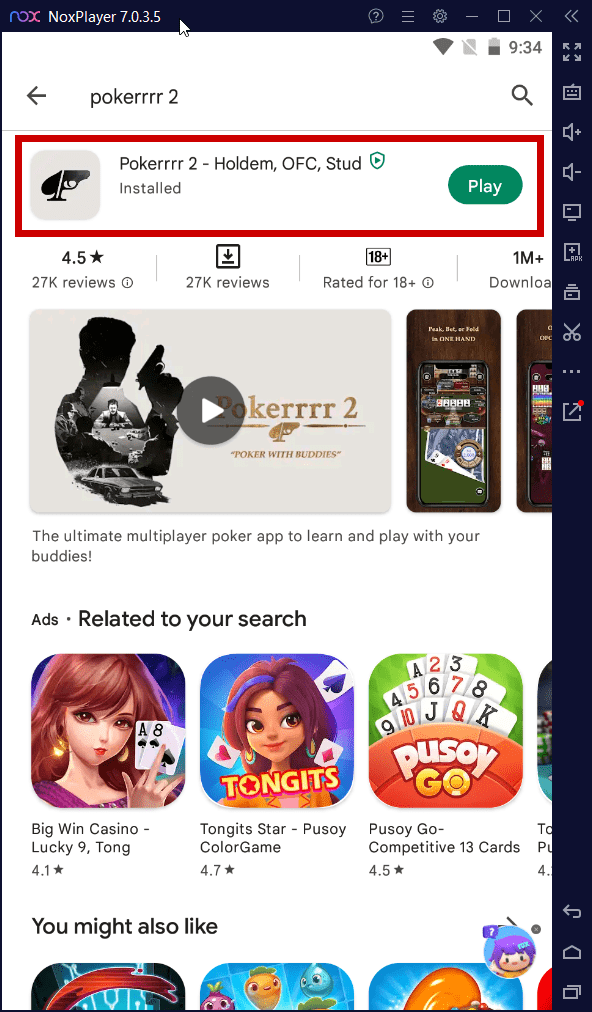The image appears to be a screenshot of a mobile device showing the app store page for a game. At the top, there's a blue bar with the text "ROX" followed by a company logo. The top bar also includes text "Knox Player, 7.0.3.5" and several icons: a question mark, three lines, a tool icon, a minimize button, a square button, an X, and two left-pointing arrows. 

Centered at the top of the screen, there is the title "Poker2" written as "Pokerrr 2". Below the title, a highlighted section reads "Poker2 - Holdem, OFC Stud", along with an "Installed" status and a play button. The app logo features a spade and a gun.

The app has a rating of 4.5 stars based on 27K reviews and is rated 18+. It boasts over 1M downloads. Below this information, there's a section with a play button to watch a trailer of the game, along with two additional game images.

Further down, an area for ads related to the search is present, showcasing other casino games like Big Win Casino, Lucky 9, Tonight Star, Pusoy Color Game, and Pusoy Go. Each ad includes relevant images, such as a woman holding cards and an image of playing cards for Pusoy Go.

Finally, a "You might also like" section is visible, featuring three more game recommendations, although details are partially obscured.